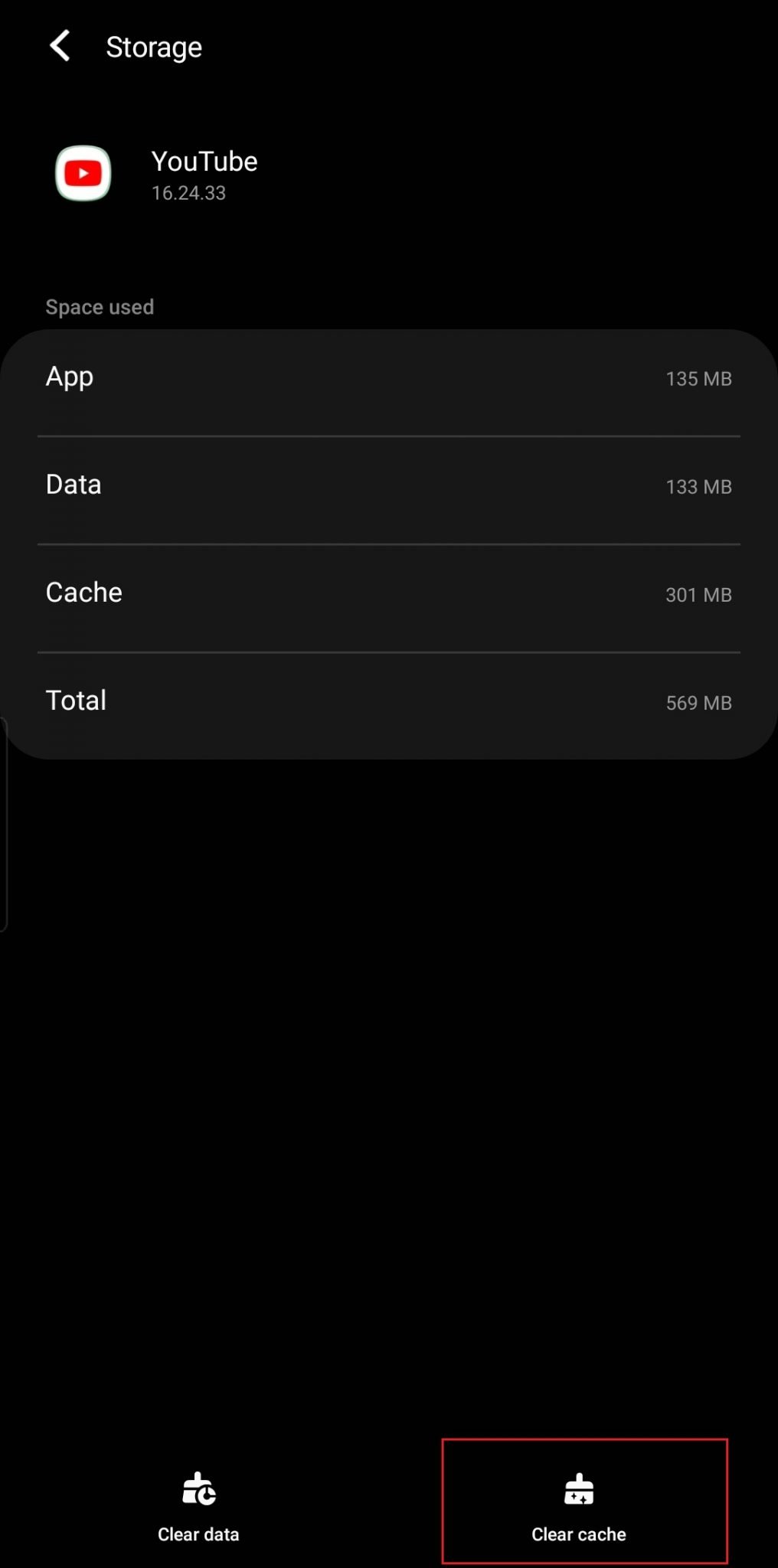The image depicts a screenshot of a screen from what appears to be a storage management application with a black background and white text. On the left-hand side, an arrow icon is present, indicating a navigation possibility. At the top of the screen, a YouTube icon is displayed alongside the word "YouTube."

Below the YouTube heading, the words "Space Used" are clearly visible. Three light gray rectangles provide detailed storage breakdowns for the YouTube application:
1. The first rectangle indicates "App" with a size of 135 MB.
2. The second rectangle lists "Data" as occupying 133 MB.
3. The third rectangle shows "Cache" taking up 301 MB.

In total, the storage used by the YouTube application is 569 MB, as stated at the bottom of this section.

Towards the bottom of the screen, there are two buttons. The first button reads "Clear Data" and features an icon of a broom with a clock in front of it. The second button is labeled "Clear Cache," accompanied by a house icon. This "Clear Cache" button is prominently highlighted with a red rectangle surrounding it, making it stand out from the rest of the elements on the screen.